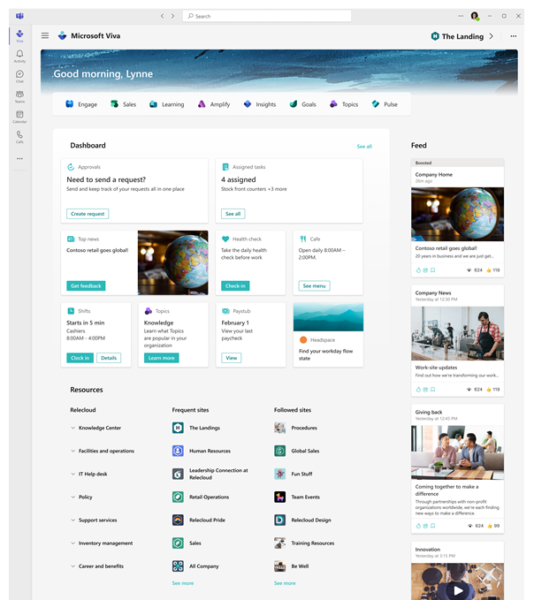Screenshot of a Microsoft Viva Web Page

This detailed screenshot captures the interface of Microsoft Viva, a web-based application. In the upper left corner, the Microsoft Viva logo is prominently displayed. Directly below the logo, a vertical menu with six navigational options is visible, alongside a menu button at the bottom for further actions.

Adjacent to the vertical menu, a horizontal hamburger menu sits just to the right of the Microsoft Viva logo, indicating additional options. At the top of the interface, a search bar is easily accessible for users to find specific content or information.

A warm greeting, "Good morning, Lynn," headlines the main content area, which appears to be a personalized dashboard landing page. Below this greeting, several key sections are listed: Engage, Sales, Learning, Amplify, Insights, Goals, and Topics. These sections likely offer quick access to various features or information areas within the platform.

To the right, a news feed provides the latest updates and relevant articles, while additional dashboard functionalities, such as a request submission feature, are also present. The overall layout and small font size indicate that the page is optimized for desktop viewing.

In the upper right corner of the interface, the user’s profile picture is situated next to the minimize, fullscreen, and exit buttons, providing easy access to user settings and window management. The detailed structure and content suggest that Microsoft Viva is potentially a comprehensive work platform designed to centralize various professional tools and information.